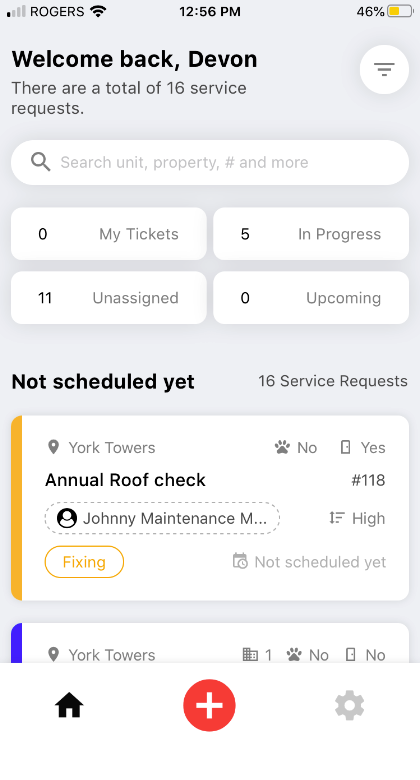The image features a user interface display set against a light blue background. At the top of the screen, it shows the network provider "Rogers," the current time "12:56 p.m.," and a battery level at "46%." The text "Welcome back, Devon" is prominently displayed.

Beneath this greeting, it is noted that there are a total of "16 service requests." To the right, there is a white circular icon with three horizontal blue lines. Below this icon, a search box is present, and below the search box, there are four small white boxes displaying ticket information:

1. **My Tickets:** 0 unassigned, 11 in progress, 5 upcoming, 0 not scheduled.
2. **Service Requests:** 16.

Further down, there is a larger white box with a yellow strip on the left. This section details a specific task: "York Towers Annual Roof Check," assigned to "Johnny Maintenance." The task is tagged as "Fixing" in a yellow box. At the top, there are options "No" and "Yes," and other details include "Number 118," "Priority: High," and it is "Not Scheduled Yet."

Another white box with a blue strip on the left mentions "York Towers," with details "Priority: 1," and has options "No" and "No." At the bottom of the screen, there is a black house icon, a red circle with a plus sign, and a small gray cog icon indicating settings.